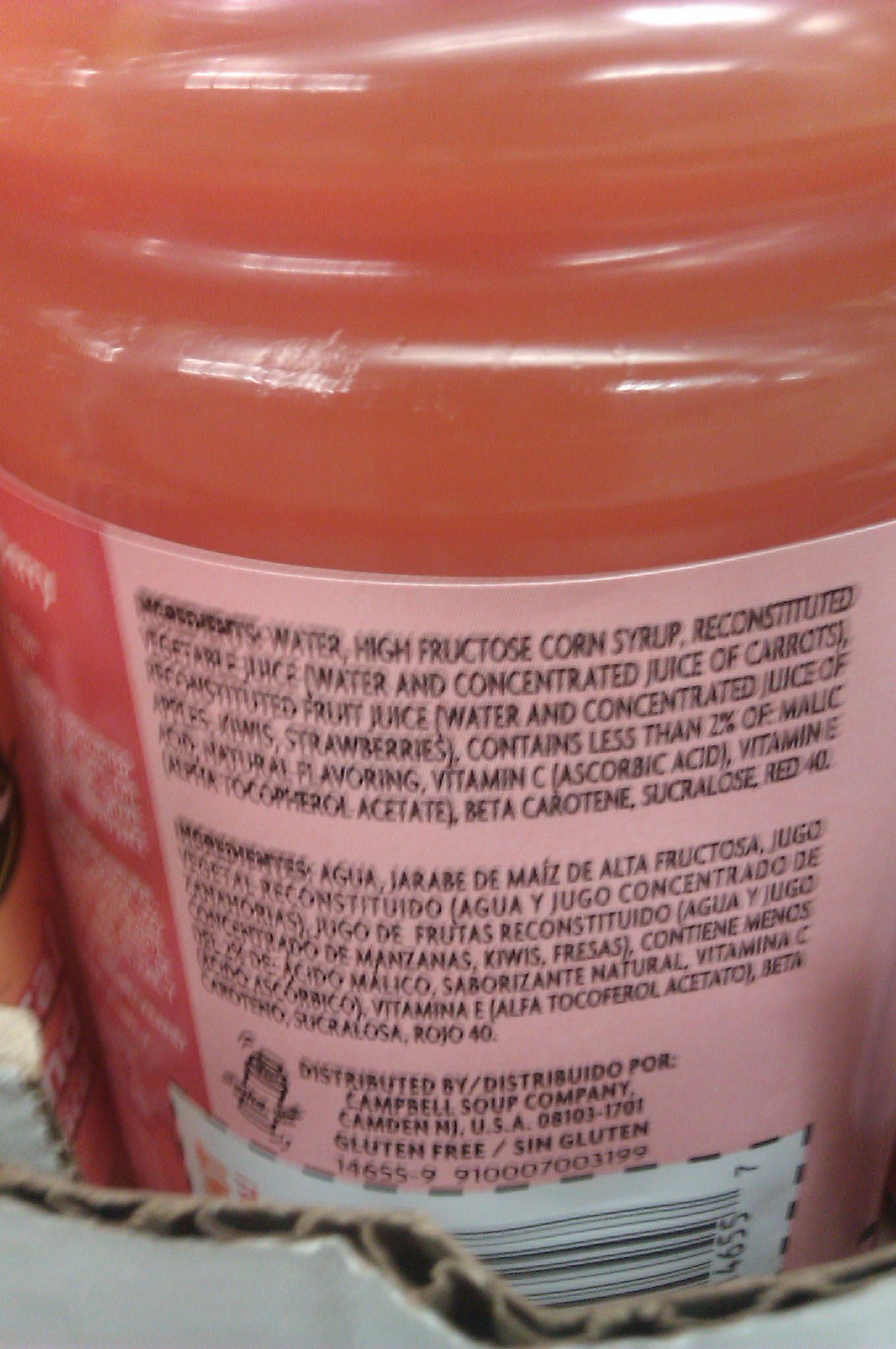Captured from the perspective of the camera, the image showcases a clear bottle with a distinctive two-tone pink label. The label features a darker pink on the upper portion and a lighter pink band around the bottom. Through the clear plastic of the bottle, a pink liquid—presumed to be juice—is partially visible. Although the image is somewhat out of focus, the lighter pink section of the label reveals a list of ingredients, including water, corn syrup, and a blend of various juices such as carrot, apple, kiwi, and strawberry concentrates. Additional ingredient information is also provided, though not entirely legible. The bottom section of the label includes distribution details indicating the product is handled by Campbell's Soup Company, located in Camden, New Jersey. This section also features further contact information and labeling specifics, along with a white box containing a barcode.